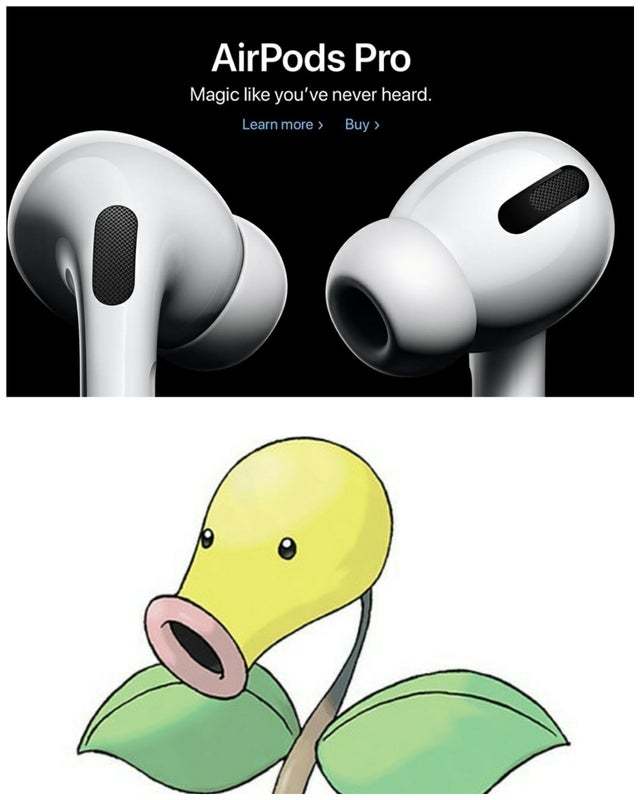This meme consists of two images arranged vertically. The top image has a black background featuring white text that reads "AirPods Pro" followed by "Magic like you've never heard." Below that are blue clickable text links with arrows labeled "learn more" and "buy." Dominating the majority of this image are close-up views of the left and right AirPods Pro, characterized by their white exterior and distinct black cylindrical sections on the side. The bottom image draws a visual comparison, showing a yellow flower with green leaves that somewhat resembles the shape and form of the AirPods Pro. The flower's head is positioned similarly to how the AirPods are aligned, reinforcing the humorous analogy. This meme humorously likens the appearance of the AirPods Pro to a character from Plants vs. Zombies, blending elements of both product advertisement and playful imagery.